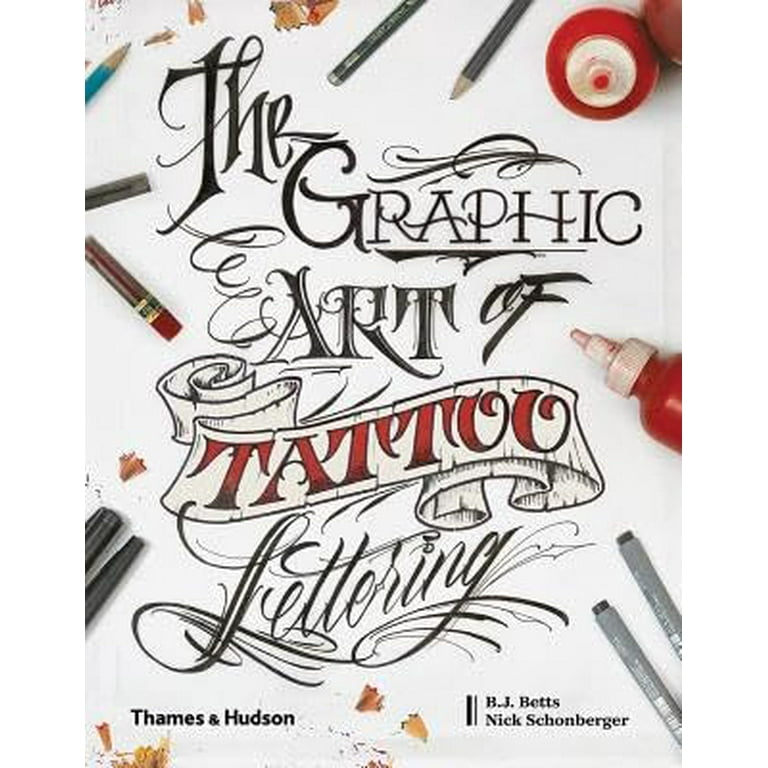This portrait-oriented image is likely the cover of a book titled "The Graphic Art of Tattoo Lettering." The text is intricately designed with each word in a different style of elaborate and ornate lettering. The words "The Graphic Art of" are in black, all different styles, and all caps. The word "tattoo" is prominently displayed in red on a white ribbon. Below, the word "lettering" reverts to a more elaborate black font with capitalized first letters. Against a white or cream-colored background, the cover features various artist tools: pencils and pens along the edges, two gray pen ends in the bottom left corner, a bottle of red ink in the right center, another bottle at the top right, and a blue pencil in the top left. At the bottom left corner is the publisher's name, Thames and Hudson, and the bottom right corner lists the authors, B.J. Betts and Nick Schoenberger.